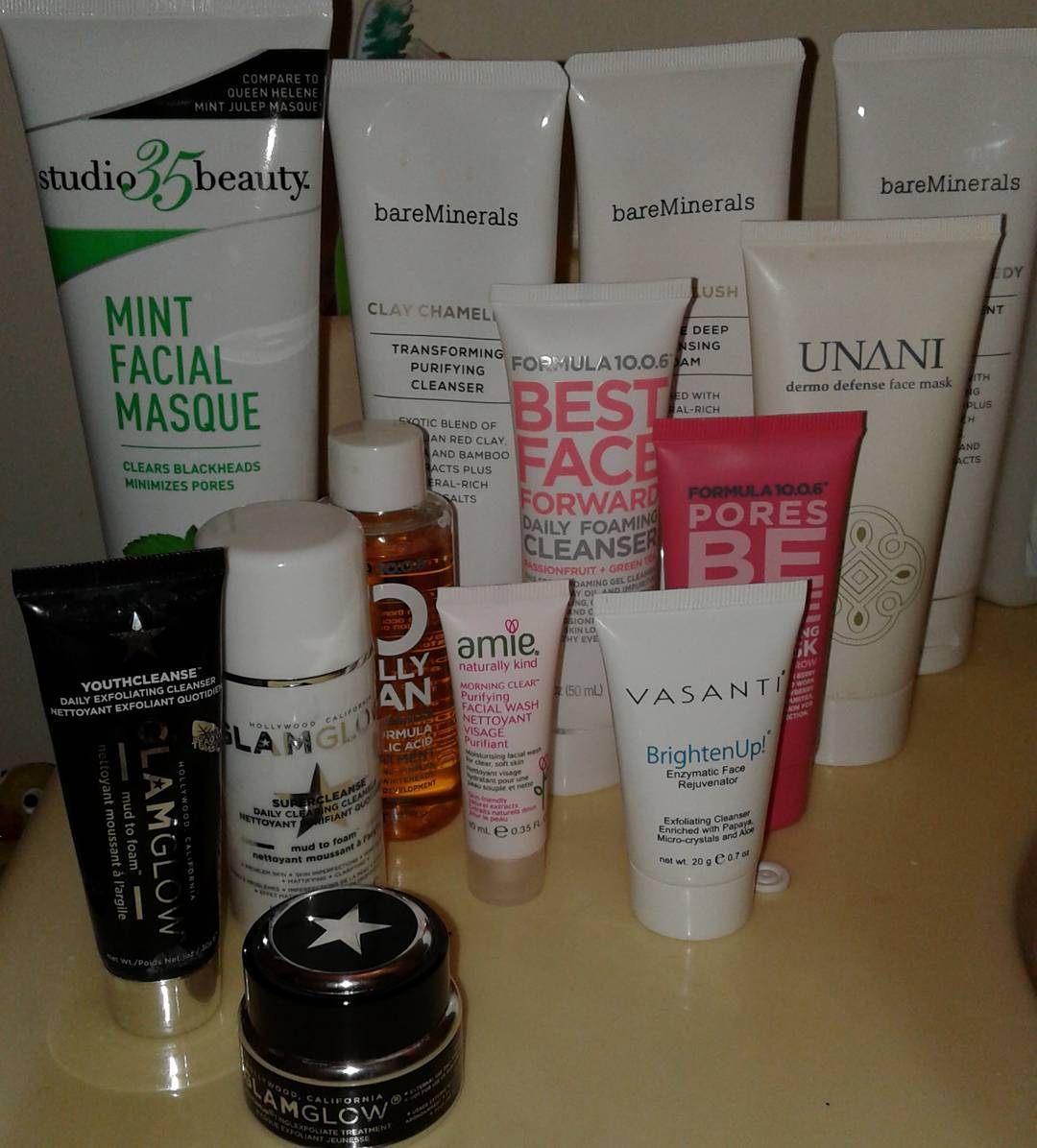In this image, an array of skincare products is neatly displayed on a light tan tabletop. At the forefront, a small black container with a white star logo prominently stands out. Just behind it, a black bottle labeled "Youthful Cleanse" in white text is visible, accompanied by additional text below. To its right, there's a small white bottle with a matching white cap.

Continuing to the right, a tiny bottle with the brand name "AMIE" is marked with pink and black text. Adjacent to this is another white bottle labeled "Visanti Brighten Up," also small in size. Positioned behind these items is a pink bottle, flanked by two more white bottles. 

Further back, a clear plastic bottle containing a brownish-orange liquid, capped in white, can be spotted. The rear row features the largest bottles, starting with one on the left branded "Studio 35 Beauty" with "Mint Facial Mask" highlighted in green text. Completing the lineup are three white bottles with the brand "Bare Minerals" embossed in black text, accompanied by various labels underneath. This composition showcases a diverse selection of skincare products lined up in meticulous order.